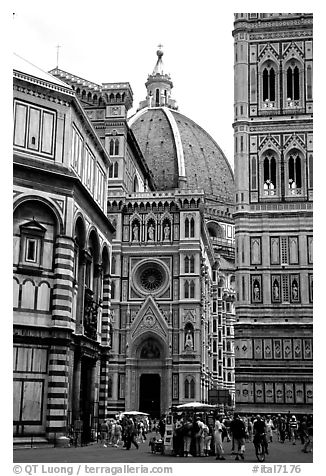This black and white photograph captures a bustling street scene in a likely European city, featuring a mix of intricate architectural styles. Dominating the center of the image is a large, temple-like structure, reminiscent of a cathedral or basilica, with a grand dome topped by a steeple and cross. Flanking the central building are two tall, ornate towers adorned with statues in their archways. The street below is alive with activity, showcasing numerous pedestrians, some of whom appear to be interacting with vendors at booths set up along the street. The overall scene provides a vivid depiction of the city's architectural grandeur and the daily life of its inhabitants.